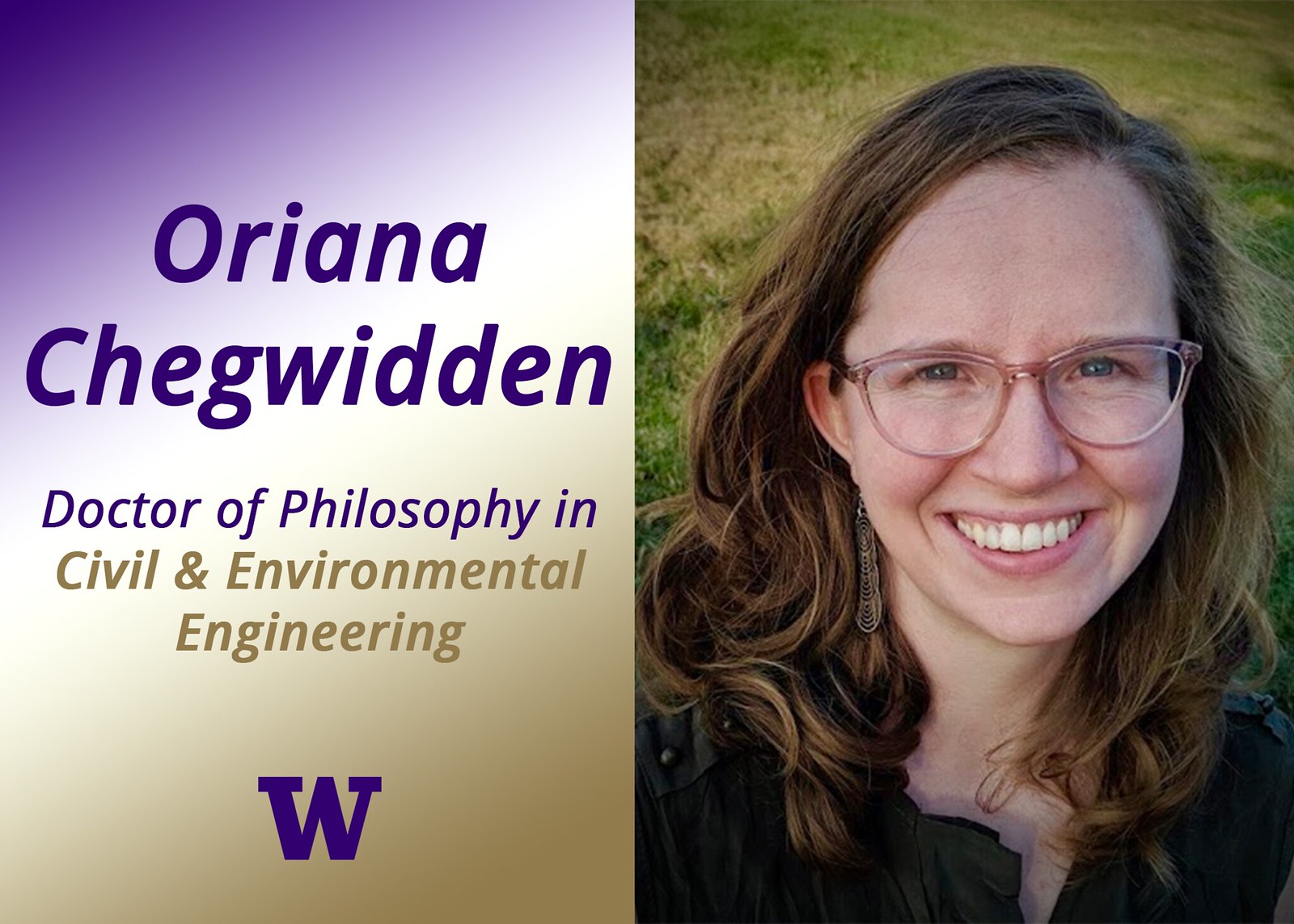The image features a rectangular layout divided into two parts. The left side showcases a background gradient transitioning from light purple to gold, with the name "Oriana Chegwidden" prominently displayed in bold purple text at the top. Beneath her name, also in purple text, it reads "Director of Philosophy." The text then changes to gold, indicating her specialty as "Civil and Environmental Engineering." At the bottom, there is a purple "W," signifying Washington University. The right side contains a portrait of Oriana Chegwidden. She is smiling and has pale white skin. She has light brown, somewhat curly hair that is around shoulder length. Oriana is wearing pink glasses and a black top, along with a long dangling earring visible on her right ear. Behind her is a backdrop of various shades of green grass, contributing a natural element to the image.